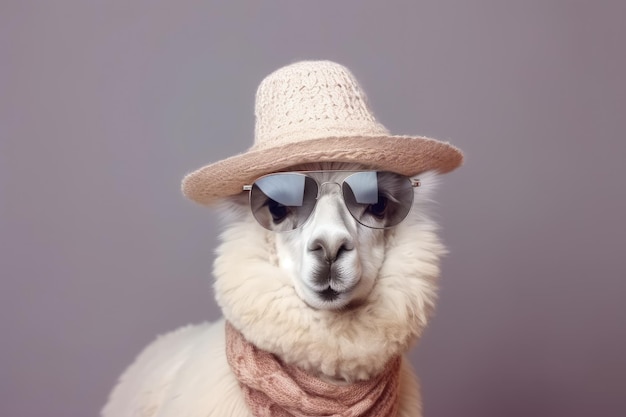This photograph features a white, fluffy animal, likely a sheep or llama, adorned with several human accessories that give it a whimsical and anthropomorphic appearance. The animal, whose ears are not visible, is captured in a portrait style, facing directly into the camera. The focus is primarily on its face, which is centered in the frame. It wears a crocheted or straw fedora-style sun hat that appears to have a hint of pink, large smoky sunglasses reflecting the studio lights, and a dusty pink knitted scarf around its neck. The background of the image is a plain gray, providing a neutral setting that highlights the animal's unique attire and fluffy white coat.